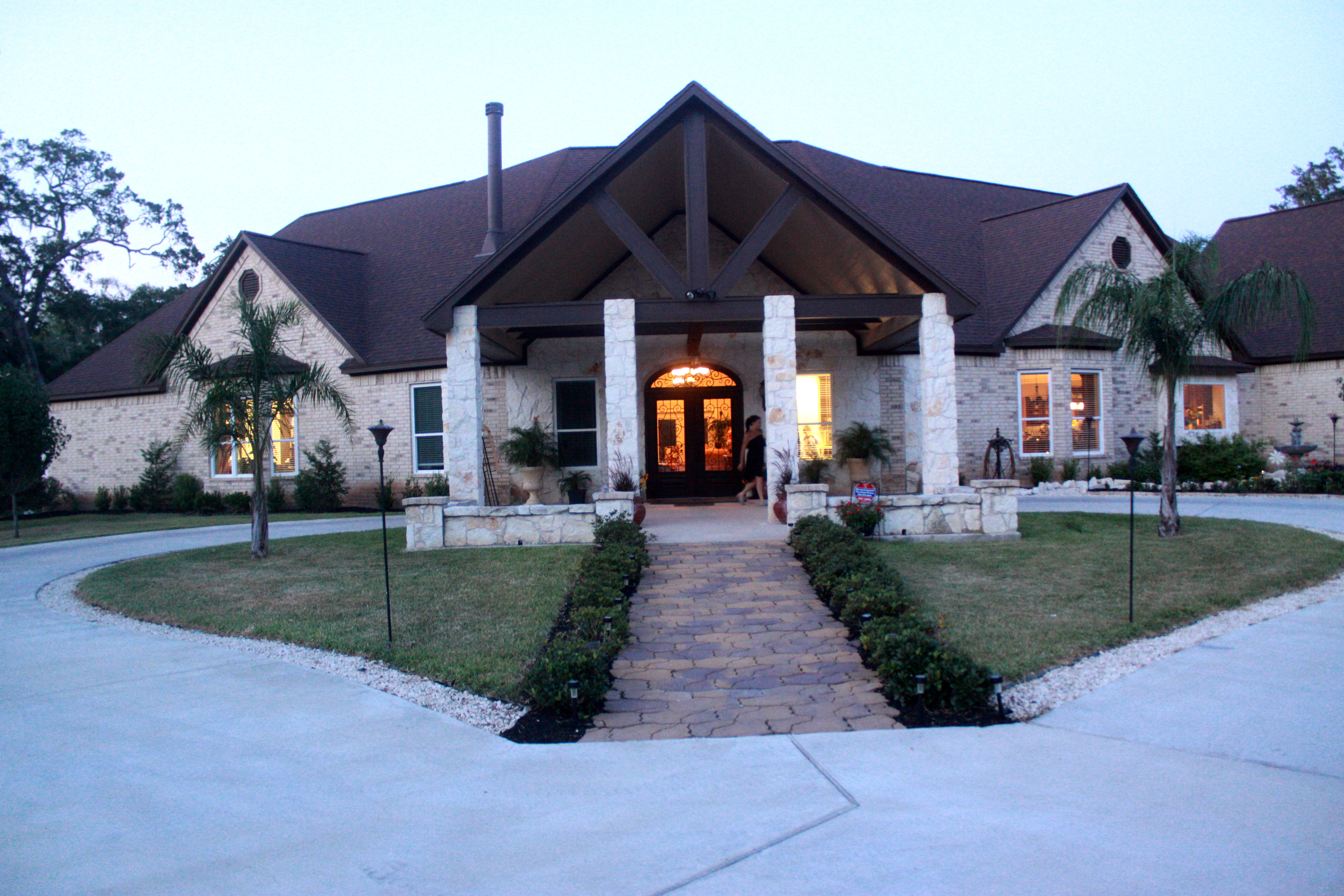The image depicts a large, light brown brick building, possibly a hotel or a substantial house, dominating the central and upper portion of the scene with a dark brown, multi-faceted roof. The building features prominent rectangular columns that support an overhang where a circular, light gray stone driveway encircles a central patch of grass. This circular driveway is situated in the foreground, and viewers look down a red stone walkway flanked by low hedges and bushes. Towards the top of the walkway, near a grand front door illuminated from within, stands a woman in a dress. The overall setting is outdoors, seemingly in the middle of the day under a pale blue sky, with additional trees, including palm trees, visible in the background, adding a touch of lush greenery to the scene.